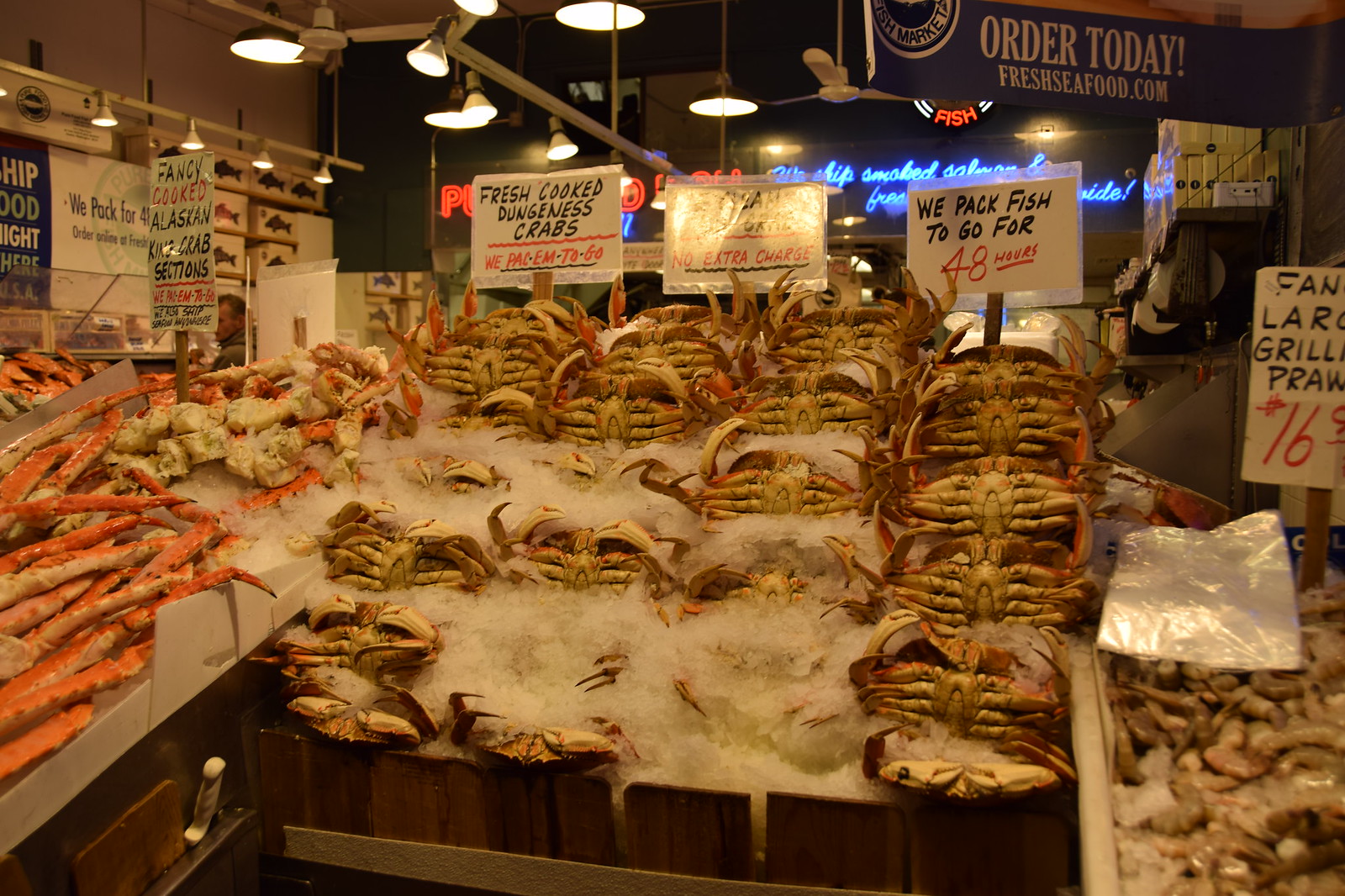The image depicts a bustling seafood market brimming with fresh seafood. Prominently displayed at the top of the scene is a blue banner that reads, "Order Today! FreshSeafood.com" in white letters. Fluorescent lights hang from the ceiling, totally illuminating the vibrant display below. 

In the foreground, there are large bins filled with ice, showcasing a variety of seafood including shrimp, crab legs, and enormous whole crabs; the crab legs, particularly striking in their bright orange color, are stacked to the left. The centerpiece consists of several rows of crabs, arranged four to five deep, some of which are nestled in ice.

Three key signs are visible. On the left, a sign states, "Fresh-Cooked Dungeness Crabs, We pack them to go." The middle sign is partially obscured by glare but is discernible, with the legible part mentioning, "No extra charge." The rightmost sign announces, "We pack fish to go for 48 hours." Additionally, peeking from the right edge of the picture, there's signage that reads, "Fancy Cooked Alaskan King Crab."

Neon signs add a splash of color to the otherwise industrial setting, despite being unreadable. This detailed and lively arrangement vividly conveys the market’s emphasis on fresh, high-quality seafood, ready to be packed for customers on the go.